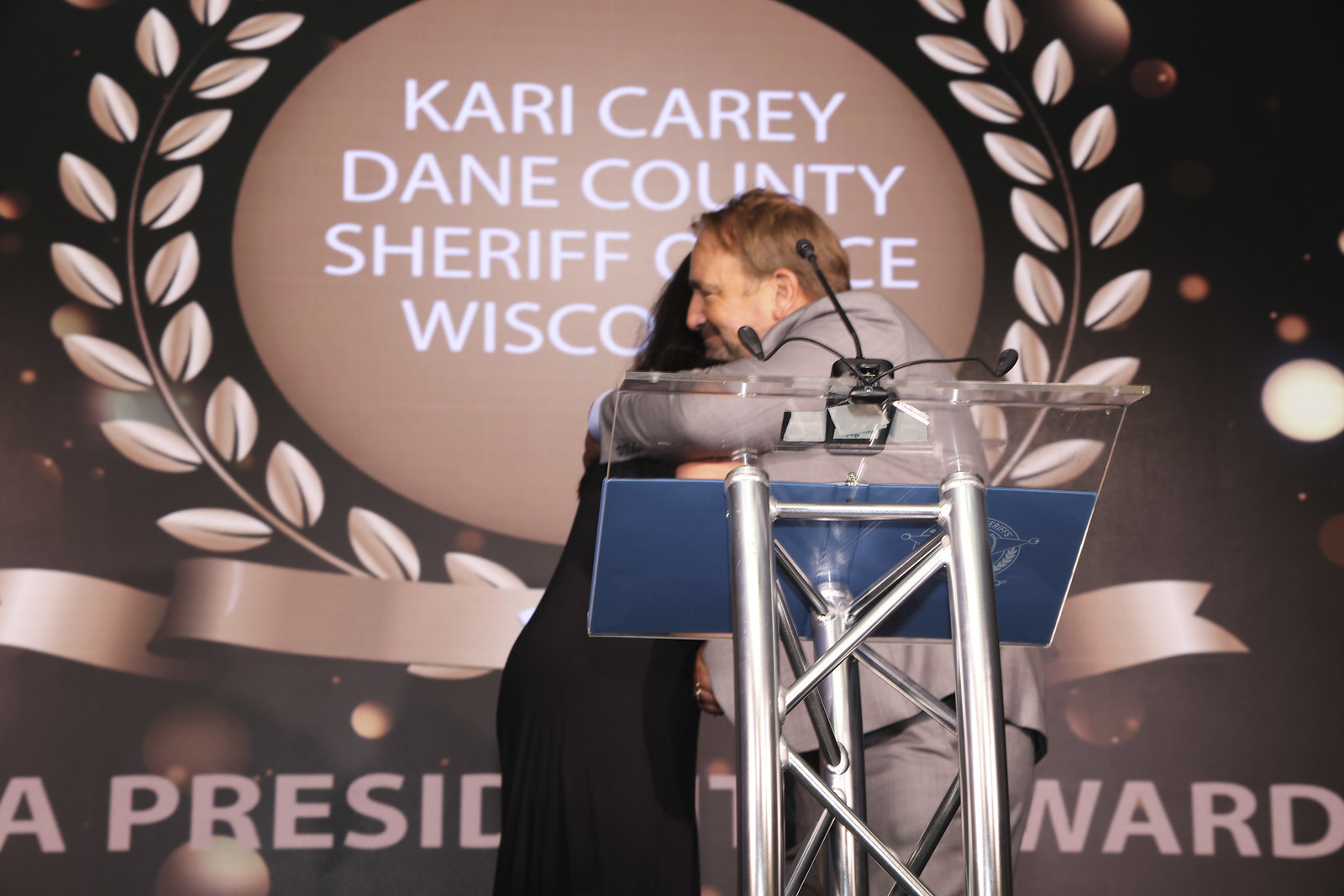In this image, we see a man and a woman hugging warmly behind a podium, suggesting the setting is an award ceremony. The podium has a unique composition with a silver metal frame and a clear, glass rectangle for the speaking surface, complemented by three black microphones at the top. A dark blue horizontal rectangle, possibly an open portfolio with an insignia, adorns the podium. 

The backdrop features a large circular banner with the names "Kari" (spelled K-A-R-I) and "Carey" (spelled C-A-R-E-Y), set against a tan background. The banner indicates the Dane County Sheriff's Office, Wisconsin, and includes a decorative design of branches with leaves around it. The bottom of the banner mentions a "presidential award," although the city name is partially obscured by the hugging figures.

The man, wearing a gray suit, has short, light brown or dirty blonde hair and a beard or goatee. The woman, dressed in a black dress, is mostly hidden behind him, with only her hair visible. The dark background of the image contrasts with the highlighted lettering and design elements, making the text and insignia stand out clearly.